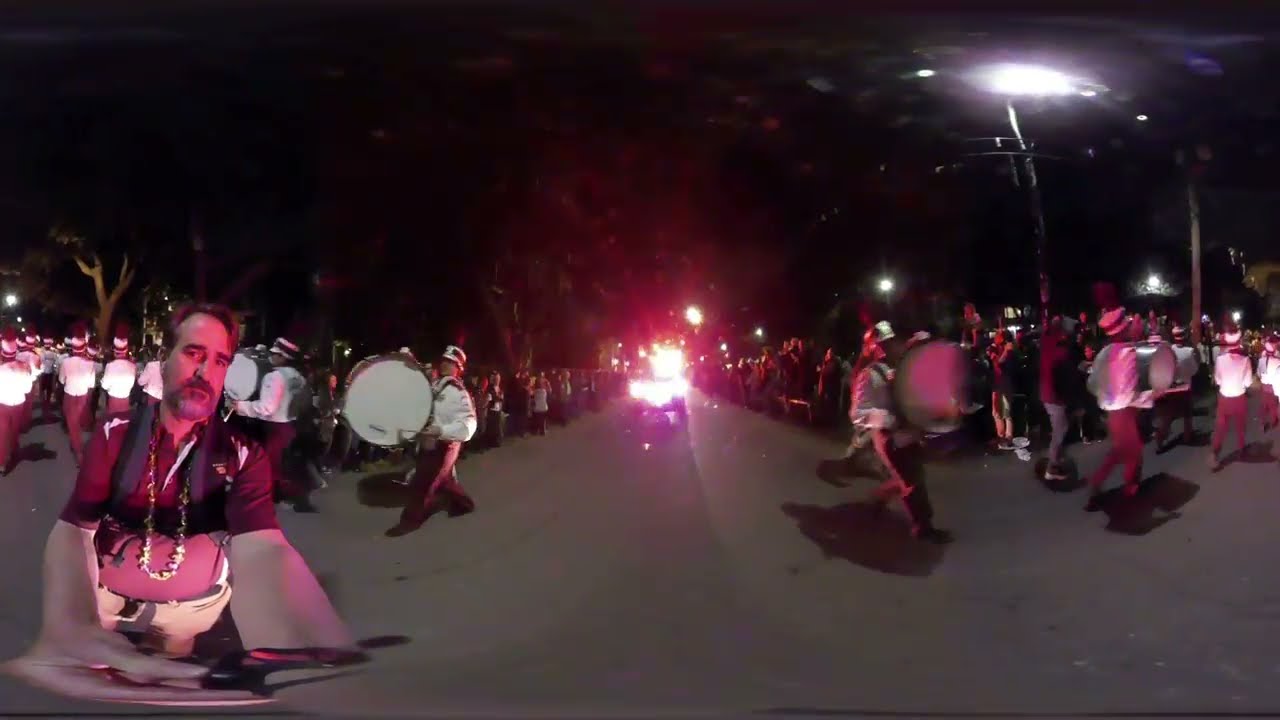This image, captured at nighttime on a dark grey cement street under a pitch-black sky, features a lively marching band parading through an outdoor public area. The band members, adorned in red or magenta pants, white long-sleeve shirts, and white caps with red feathers, are marching while holding large drums. The photograph has a distinctive fisheye effect, making the edges appear warped while the center remains normal. On the left side of the image, a man with short brown hair and a goatee is seen using a selfie stick to take a picture of himself. He is dressed in a red, short-sleeved polo shirt and beige khaki pants, with a backpack on his shoulders. Behind him, the brightly lit street reveals more members of the marching band and other people lined up along the sides. A car with its headlights on can be seen approaching from the background, adding to the bustling, nighttime atmosphere.